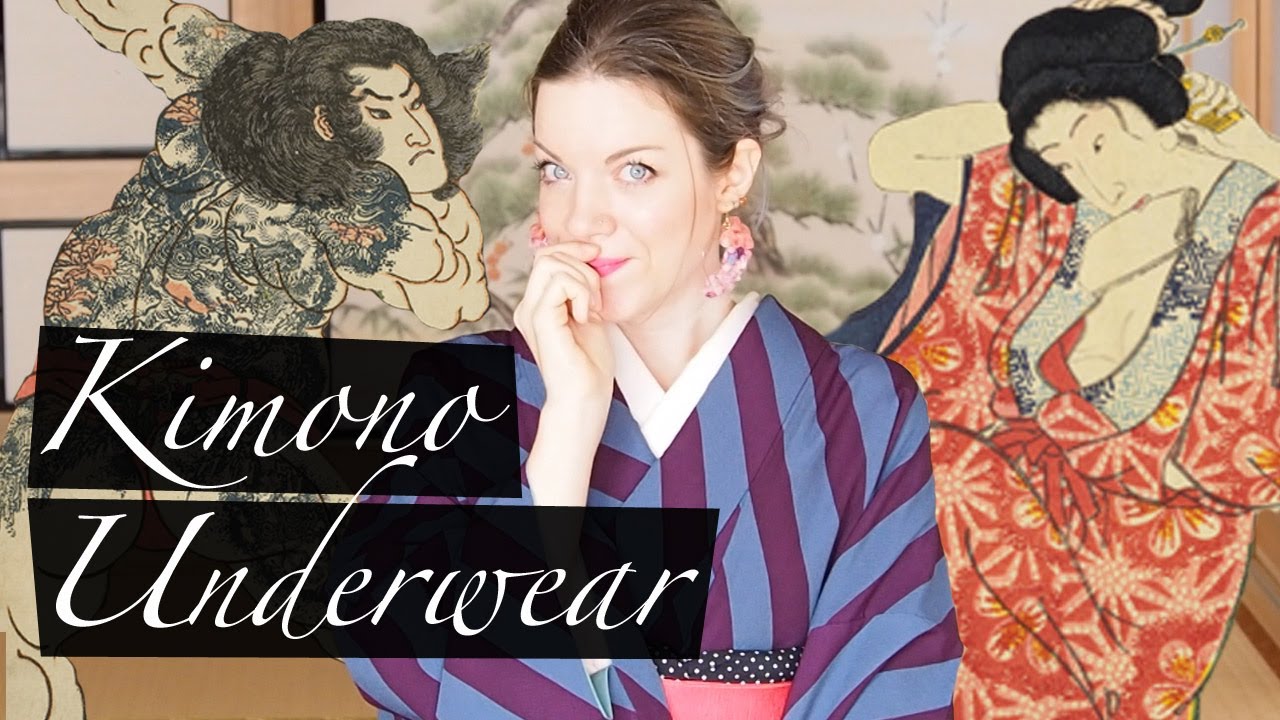This image is an advertisement for kimono underwear, featuring a Caucasian woman with light brown hair, dark hair pulled back, and wearing dangly earrings. She is dressed in a kimono with maroon and blue stripes, a white v-neck, and a distinctive pink pocket accented with a black line featuring white dots. Her right arm is extended with her hand near her mouth. Behind her is an artistic backdrop of a Japanese-style illustration, with a depiction of a sumo warrior to her left and a woman resembling a geisha to her right. Both figures are dressed in traditional kimonos; the woman is in red and white, and the man in black, white, and red. Two black banners in front of the main figure read "kimono underwear" in white lettering. The background of the image includes a depiction of white clouds, adding a serene and cohesive element to the advertisement.